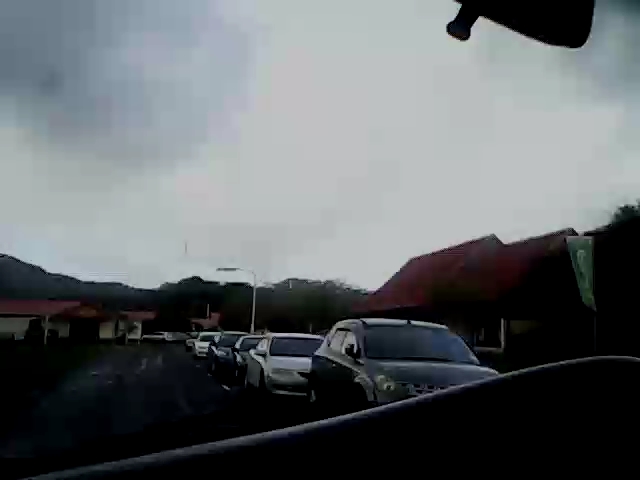The photograph, taken from inside a car through the windshield, presents a gray, overcast sky blanketing the scene. In the upper right-hand corner, part of the rearview mirror is visible, contributing to the sense of being inside the vehicle. The sky features light gray and dark gray clouds, with some pixelation giving an impression of a low quality image. The scene outside shows a row of parked cars on the right side of the road, with a mix of dark and white vehicles. Beyond the cars, rooftops of houses with red roofs are visible amidst the cloudy backdrop. Streetlights stand dormant along the road. In the distance, low hills or mountain terrain can be seen, adding depth to the background scenery. The image also captures part of the dashboard and a label on the windshield, adding to the details of the interior view.